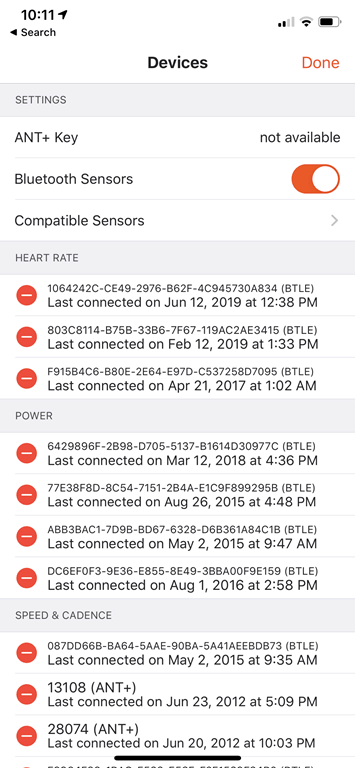**Detailed Caption:**

This screenshot appears to be from a health or fitness application, specifically showcasing various connected Bluetooth sensors used to monitor different fitness metrics. The interface displays multiple categories such as heart rate, power, speed, and cadence. 

On the left side of the screenshot, there are several bright orange indicators marked with little dashes. Each indicator seems to represent a different recorded session or a connected device. For heart rate, there are three indicators, for power there are four, and for speed and cadence, there are three each.

The timeline of data logging reveals that the user's devices were connected intermittently over the years, with notable timestamps including:
- June 12, 2019
- February 12, 2019
- May 12, 2018
- April 21, 2017
- August 26, 2015

The details suggest that the user checks these metrics periodically, possibly for tracking their fitness progress over time. Overall, the screenshot organizes a comprehensive overview of the user’s recorded fitness data, albeit in a somewhat complex and technical manner.